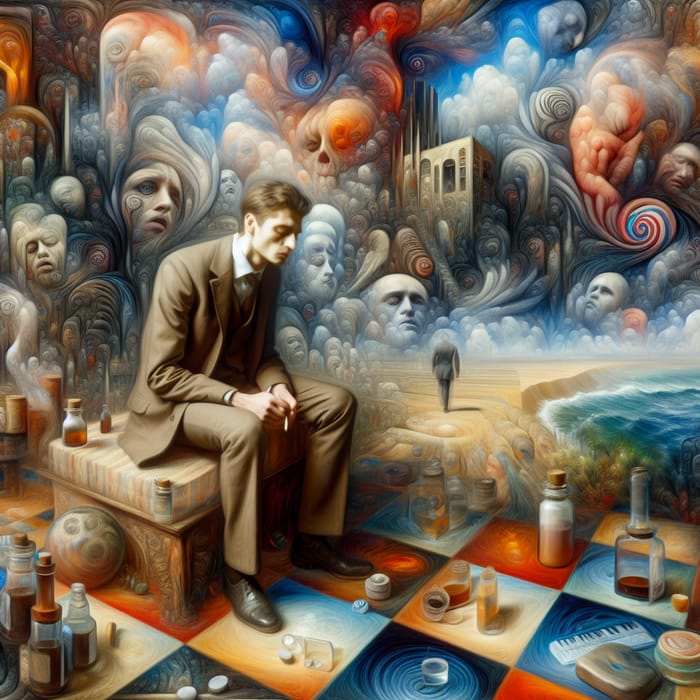The artwork, possibly an illustration or painting, depicts a solitary man seated on a bench, exuding an air of melancholy. He is dressed in a brown three-piece suit, complemented by black dress shoes, and his head is bowed as he gazes downward, a cigarette poised between his fingers resting on his lap. His short brown hair adds to his somber appearance. The ground beneath his feet is a vibrant and abstract checkerboard of squares in hues ranging from light blue, white, and brown to green and orange, littered with numerous bottles, cups, and large pills. Beside him on the bench, a bottle containing a brown liquid suggests a possible struggle with addiction. Surrounding him is a perplexing environment, with distressed faces rendered translucent above the ground and along the sealed walls, possibly symbolizing haunting thoughts or memories. Adding to the surreal scene, the ground transforms on the right side into a beachscape, where a man, also in a suit, strolls along the shore as waves crash nearby. Above, a mélange of smoke, cloud designs, and ghostly figures, some resembling skeletons or skulls, swirl in the air, further evoking themes of despair and introspection.